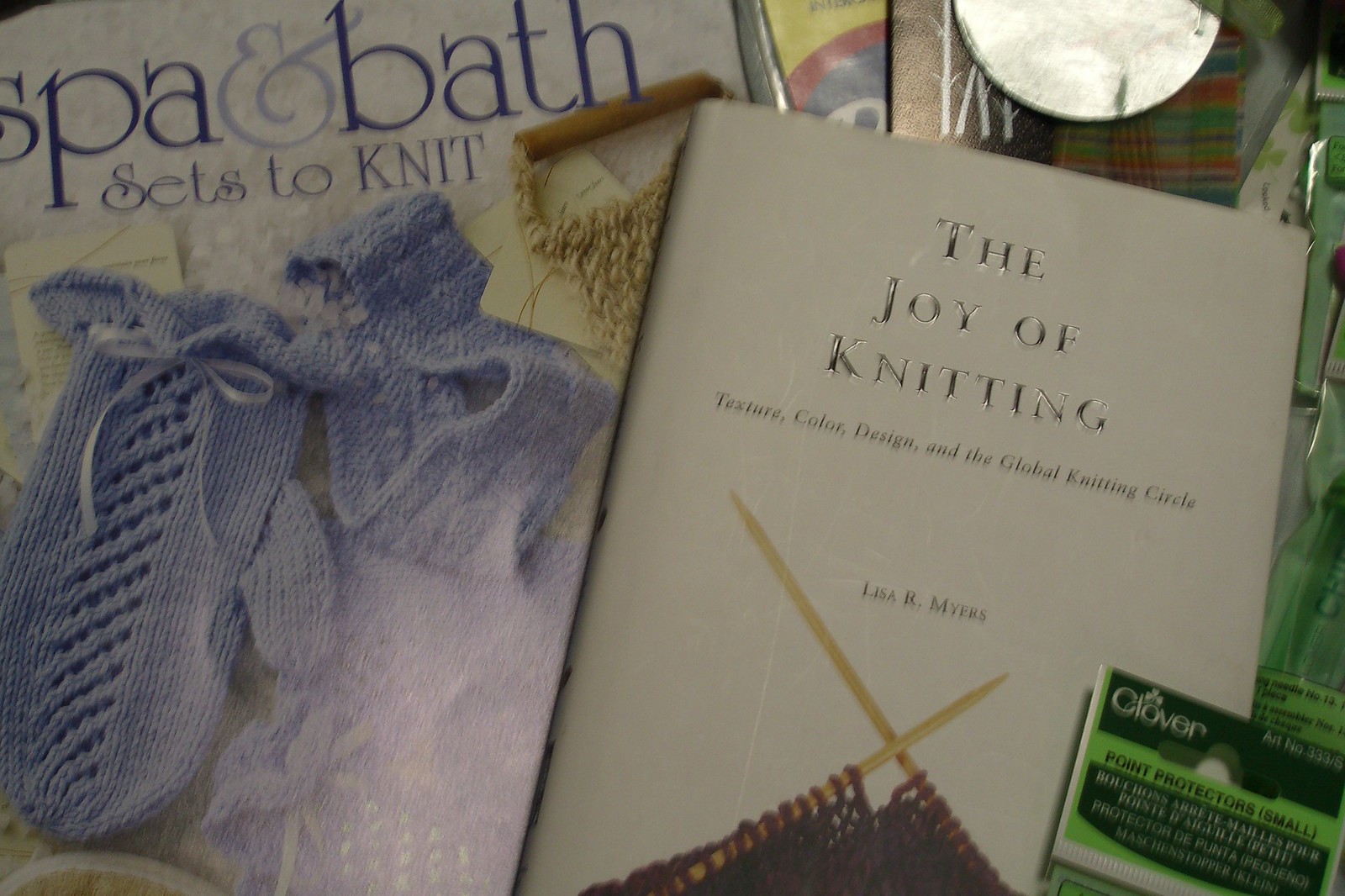The image is a color close-up photograph of a collection of books and knitting materials lying on a cluttered surface. On the left side is a booklet titled "Spa and Bath Sets to Knit," featuring an array of knitted blue socks and blue fabrics on its cover. Pressed against it is a light gray hardcover book with a metallic title that reads "The Joy of Knitting: Texture, Color, Design, and the Global Knitting Circle" by Lisa R. Myers. The book cover displays a pair of gold knitting needles with dark red thread looped around them. In the bottom right corner, a small green packet labeled "Clover: Point Protectors, Small" is partially visible, with some text too small to read. The table beneath the items appears to be cluttered with scrap paper of various colors, adding to the busy yet cozy scene.